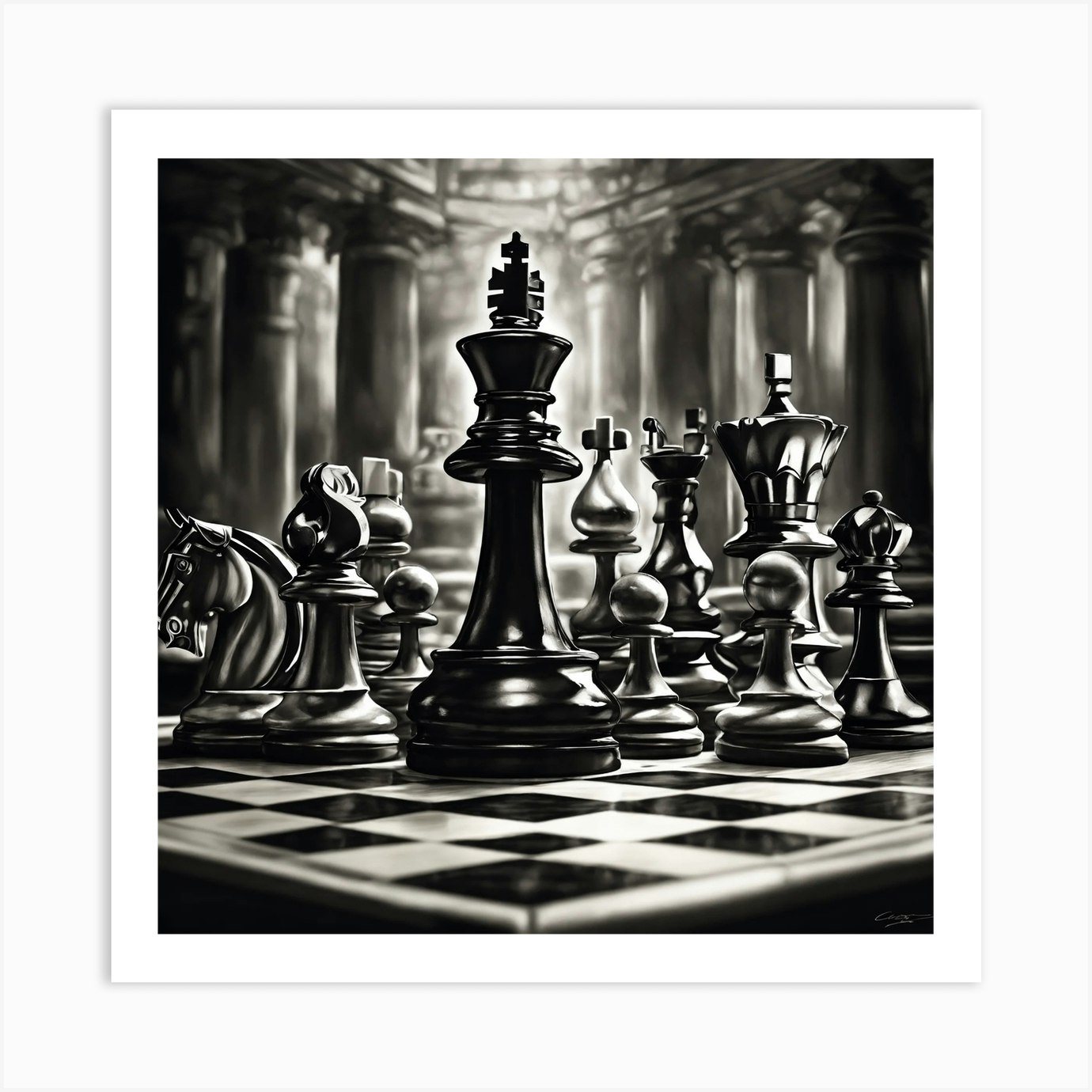This black-and-white drawing artfully depicts a realistic yet artistic representation of an oversized chessboard, dominated centrally by a large Black King piece. Surrounding it, to the left, are a knight facing left and a bishop, while to the right stand two pawns, the queen, and another bishop. The background is adorned with Greek or Roman-style pillars, lending a classical architectural touch to the scene. The chess pieces are all black but exhibit white highlights mimicking light reflection, adding to their three-dimensional realism. The perspective is eye-level with the chess pieces rather than the traditional top-down view, emphasizing the prominence and grandeur of the Black King against the lighter backdrop.